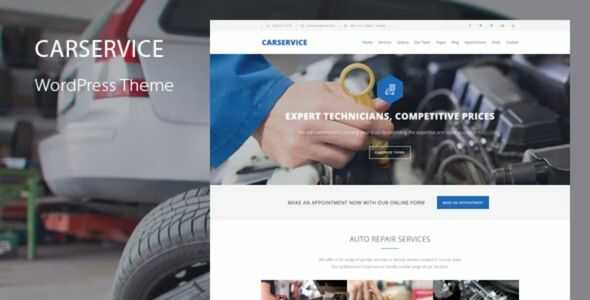This image showcases a detailed WordPress theme mock-up, specifically designed for car service businesses. The background features a faded, high-resolution photograph of the rear of a crossover SUV elevated on prominent red struts, likely indicating that the vehicle is undergoing maintenance or repair. Tires are scattered in the foreground, adding to the automotive theme.

In the upper left corner, crisp white text announces "Car Service WordPress Theme." To the right, a superimposed image reveals the layout and design of the theme. This preview highlights a typical WordPress structure with a large horizontal header image depicting a mechanic in a blue-sleeved shirt extracting a dipstick from a car engine. Overlaying this header image, white text proclaims "Expert Technicians, Competitive Prices," reinforcing the theme's focus.

At the top of the superimposed theme, "Car Service" is displayed as a single word on a white background, accompanied by a series of low-resolution, unreadable menu options arranged in a row. Below the header image, there is a gray banner featuring a noticeable blue button. Further down, a section on a white background titled "Auto Repair Services" includes an unreadable descriptive blurb. The section is followed by three truncated images aligned side by side, which are partially cut off at the bottom edge of the mock-up. Overall, this mock-up effectively presents the key elements and visual style suitable for a car service WordPress theme.